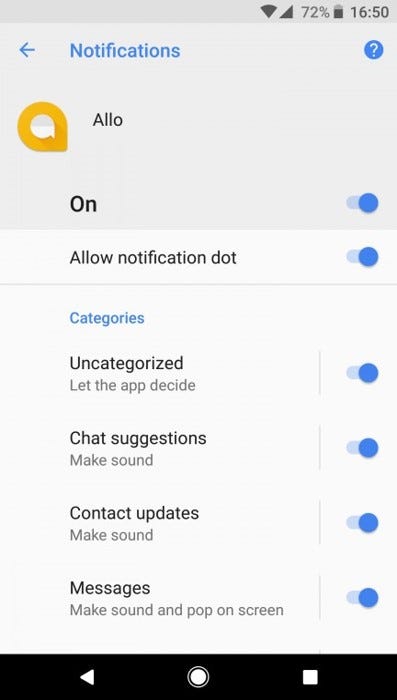This image captures the notification settings screen of a cell phone, with a light gray background that fades to a darker shade at the top. At the very top of the screen, in the darkest gray area, icons for Wi-Fi signal strength and a triangle symbol are visible, with the battery level at 72% displayed beside a dark gray battery icon. The time is shown as 16:50. The word "Notifications" is prominently displayed in blue with a left-pointing arrow beside it, and a white question mark inside a blue circle is also visible.

On the left side, beneath the top section, the text "ALLO" is present, accompanied by an orange speech bubble icon with a smaller white speech bubble inside it. Adjacent to this, the word "on" is displayed with a slider that has a blue circle slid all the way to the right, indicating that notifications are allowed. Below this, a faint gray line separates the top section from the categories section. The categories listed below all have their notification settings turned on, indicated by blue dots on the right side of the screen.